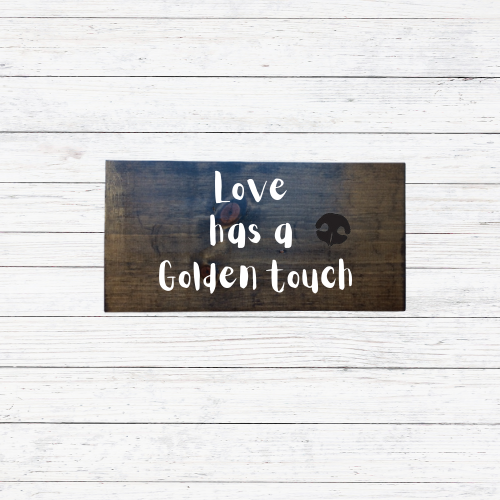The image shows a close-up of a rectangular, whitewashed wooden exterior wall composed of horizontal panels, some of which are more worn and narrow towards the center. The wall, painted white, has patches of the paint coming off, revealing a darker wood beneath. The center of the image features a small, dark brown rectangular wooden sign, approximately one and a half inches wide and just under an inch high, with a prominent knot in the middle. The sign displays the quote "Love has a golden touch" in three rows of white, handwritten-style text. Above the word "touch," there's a brown shadowy outline, which might resemble either a flower or an animal's snout. The overall dimensions of the image are roughly square, about four inches by four inches.